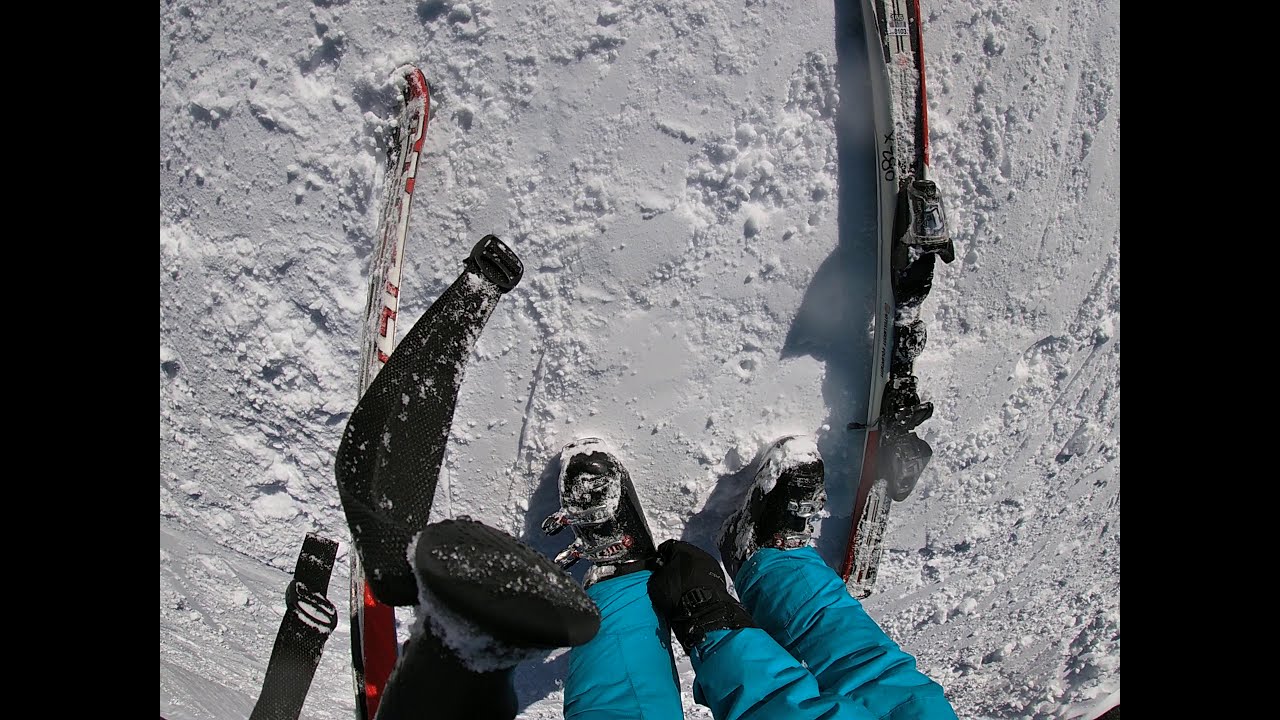In this color photograph taken from a GoPro or helmet-mounted camera, we see a close-up view of a skier standing in deep snow. The skier is wearing black snow boots with buckles, and a turquoise, retro-style snowsuit. Both feet are positioned firmly in the snow, with the two skis lying parallel to the left and right of their feet. The skier's hands, clad in black mittens, are visible—one hand is adjusting the pant leg of the snowsuit. The left hand appears to be holding both ski poles, which have black handles and straps. The entire background and ground are covered in pristine white snow, filling the frame and emphasizing the skier's gear and position.